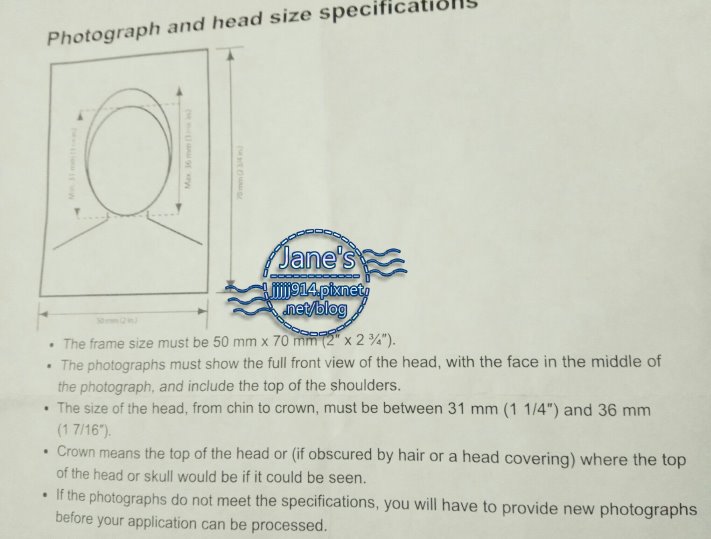The image captures a slightly angled photograph of a detailed gray information poster about passport photo requirements. At the very top left, the title "Photograph and Head Size Specifications" is prominently displayed in black lettering. Below this title, a rectangular diagram illustrates the dimensions for the photo, with arrows indicating the specific measurements for width and height. Centrally within the rectangle, black-lined ovals depict the hair and face areas, with arrows showing how the space should be utilized, including slumping lines to represent the shoulders.

Stamped diagonally across the middle of the poster is a blue logo that reads "Jane's" followed by "914picsnet.net/blog," outlined in blue with wavy lines around the text. Beneath this logo, the poster provides extensive instructions in gray letters, structured in a bullet-point format. Key points include:
- "The frame size must be 50 millimeters by 70 millimeters (2 inches by 2 3/4 inches)."
- "The photograph must show a full front view of the head with the face centered and include the top of the shoulders."
- "The head size, from chin to crown, must be between 31 millimeters (1 1/4 inches) and 36 millimeters (1 7/16 inches)."
- "If obscured by hair or a head covering, the 'crown' refers to where the top of the head would be if visible."

It is noted that any photographs not meeting these specifications will require resubmission before the application process can proceed.